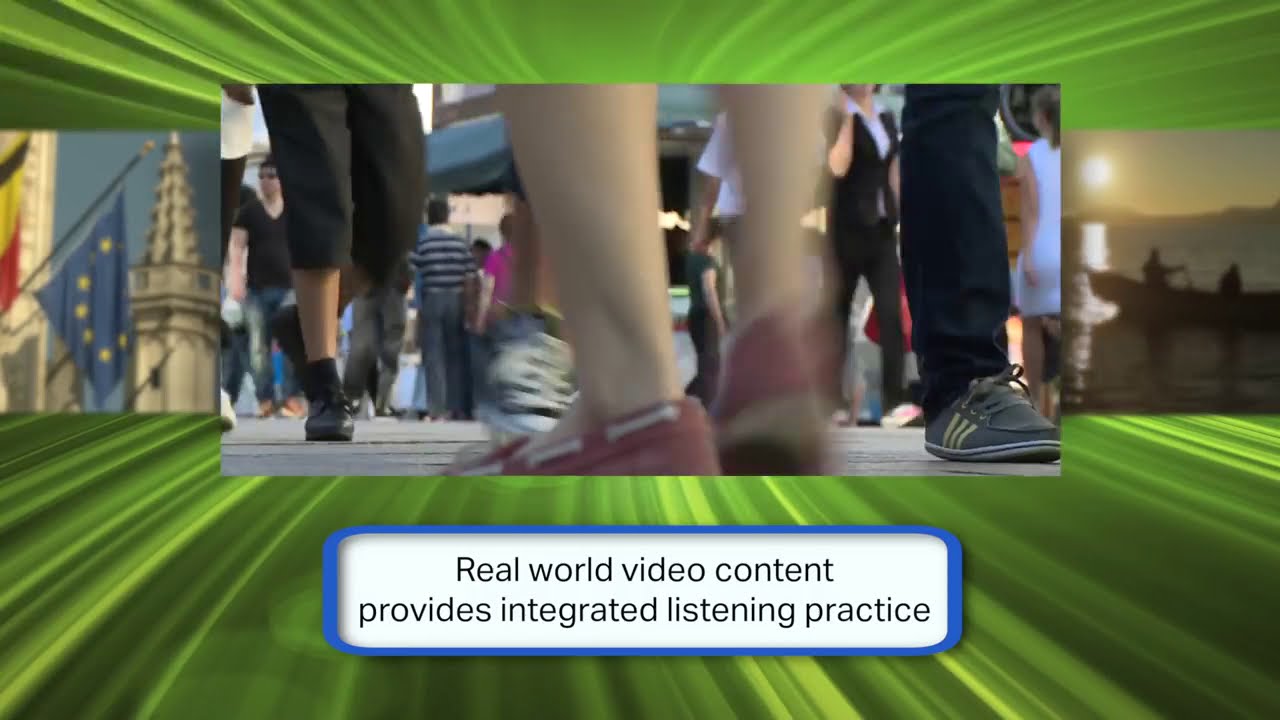The image showcases a surreal photograph that almost appears computer-generated, capturing people's legs in motion on a street, with a focus on a pair of red boat shoes in the foreground. The right leg of this figure is notably blurry, suggesting movement. The scene is set against a dynamic background of green hues and light green rays extending into the distance, evoking a Tron-like effect.

Accompanying the central image are two smaller photos positioned left and right, somewhat behind the main picture. The left photo depicts a blue flag with yellow stars in a circle, set against a white building, reminiscent of looking at a European landmark. The right photo features a serene sunset scene of two people in a rowboat on a lake, adding a tranquil counterpoint to the dynamic central image.

Below the primary photo, a white rectangular block outlined in blue contains black text that reads, "Real-world video content provides integrated listening practice," integrating the images into an educational or media context. This detailed composition not only highlights the varied footwear and movement on a busy sidewalk but also immerses it in a vivid, almost futuristic setting.